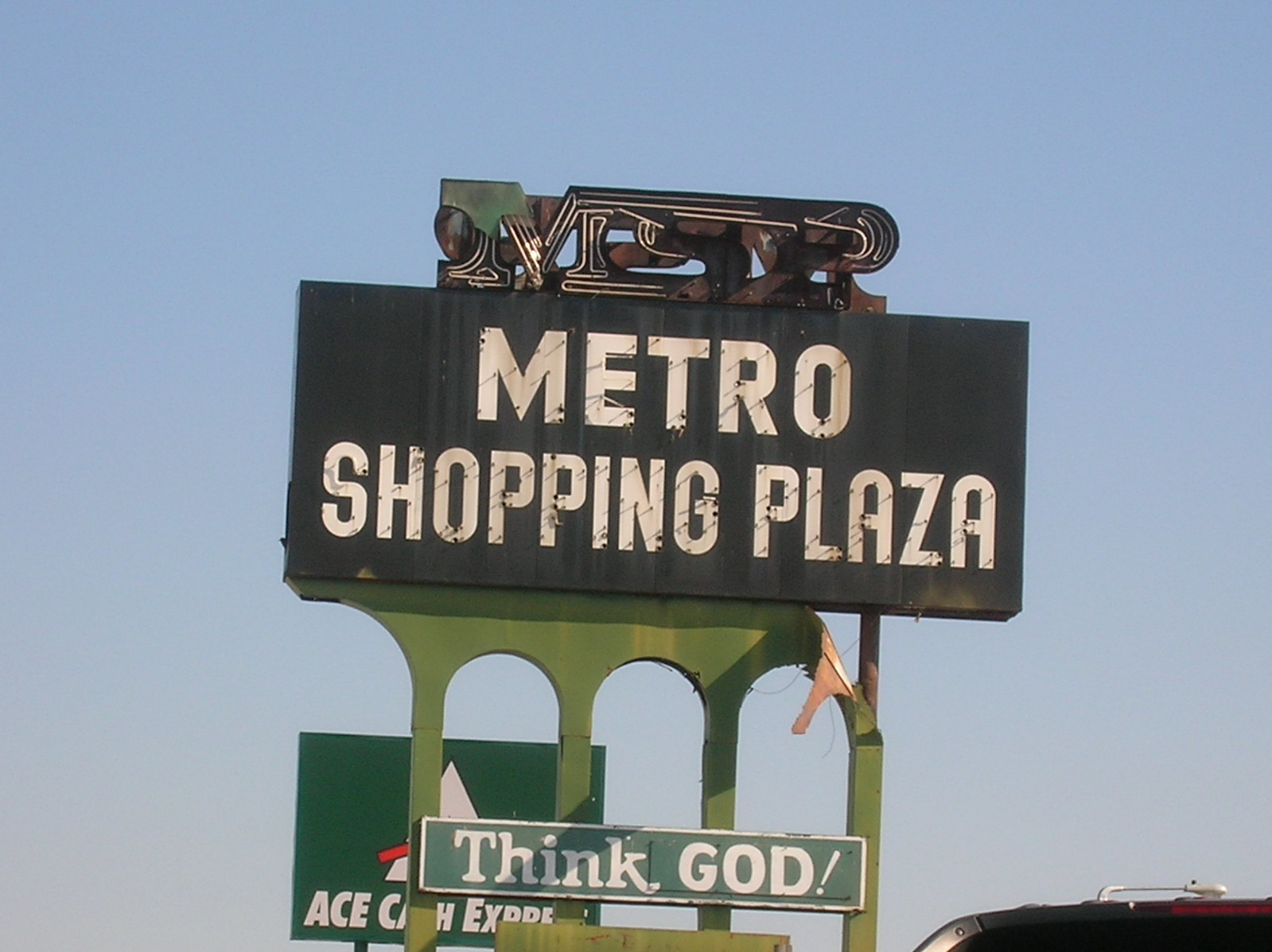A well-focused color photograph captures a tall, freestanding sign against a light blue, clear sky. The sign, which looks old and poorly maintained, serves as the marquee for the "Metro Shopping Plaza." This main portion of the sign is a black or dark green rectangle with large, white letters. The remnants of once-functioning neon lights frame the top, though they are now mostly broken, with only a hint of the letter "M" visible. Supporting the sign are four green pillars, partially covered in sheet metal shaped like arches, which are rusting and deteriorating. Beneath the "Metro Shopping Plaza" sign, a smaller green board reads "Think God!" in white text. In the lower right corner of the image, the top of a pickup truck's cab and a streetlight arm are partially visible. Behind the main sign, slightly to the left, another smaller sign for "Ace Cash Express" peeks out, with some letters obscured by the pillars. The scene suggests a somewhat neglected area, perhaps in the southern United States, given the religious signage.